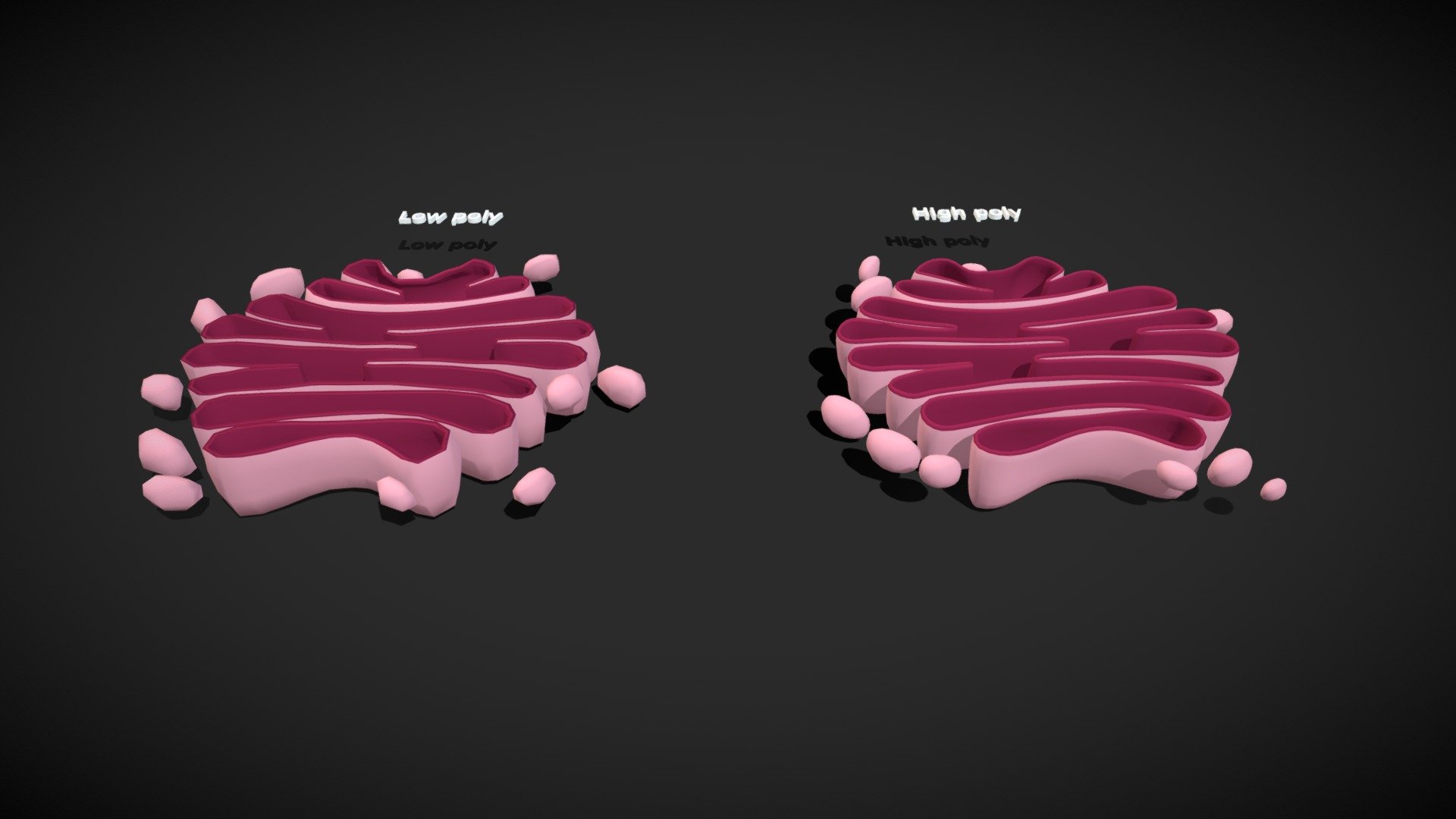The image features two 3D renders of a Golgi apparatus, each comprised of a series of pink tubular structures stacked in layers. The higher detailed render on the right prominently labeled "high-poly" in white 3D text with a shadow beneath, displays smoother, more refined edges. In contrast, the render on the left, marked "low-poly," is notably blockier and more jagged, with a similar 3D shadowed label. Both structures are colored with a gradient: light pink to almost white exteriors and deep pink interiors. They are reminiscent of deli meat slices rolled in a circular fashion, with scattered, rounded oblong shapes of light pink around them. These digital representations are set against a slate gray background that darkens towards the edges, emphasizing the centered 3D renders. The entire composition measures approximately six inches wide by three inches high.